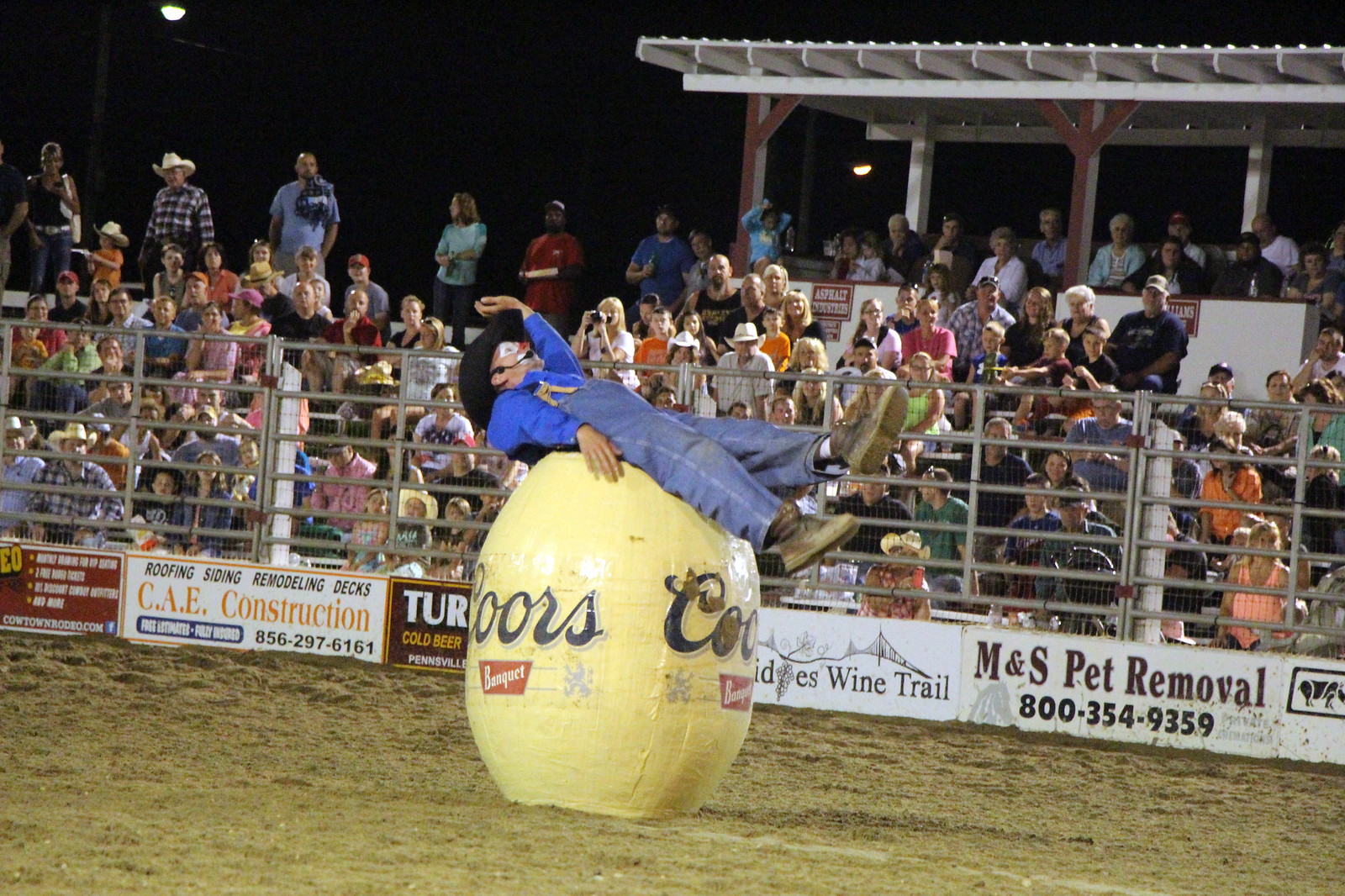In the center of this image, set in an outdoor rodeo event, a rodeo clown is prominently featured. The clown, donning blue overalls, clown face paint, a red nose, and a black cowboy hat, is perched atop a yellow barrel labeled "Coors Banquet." The ground surface is a sandy, dirt-filled arena, indicative of a typical rodeo setting. Surrounding the central figure, we see numerous details: a large crowd is gathered behind a fence or gate to the right, cheering from white stands. Above the crowd, an announcer’s booth is visible against the sky, indicating it's daylight. Advertisements line the barrier and fence, including mentions of "MS Paint," "MS Pet Removal," "Wine Trail," "Turtle Beer," "CAE Construction," and a red sign. The scene is vibrant with colors such as tan, brown, red, white, blue, gray, pink, purple, and orange, capturing the lively atmosphere of a rodeo performance.